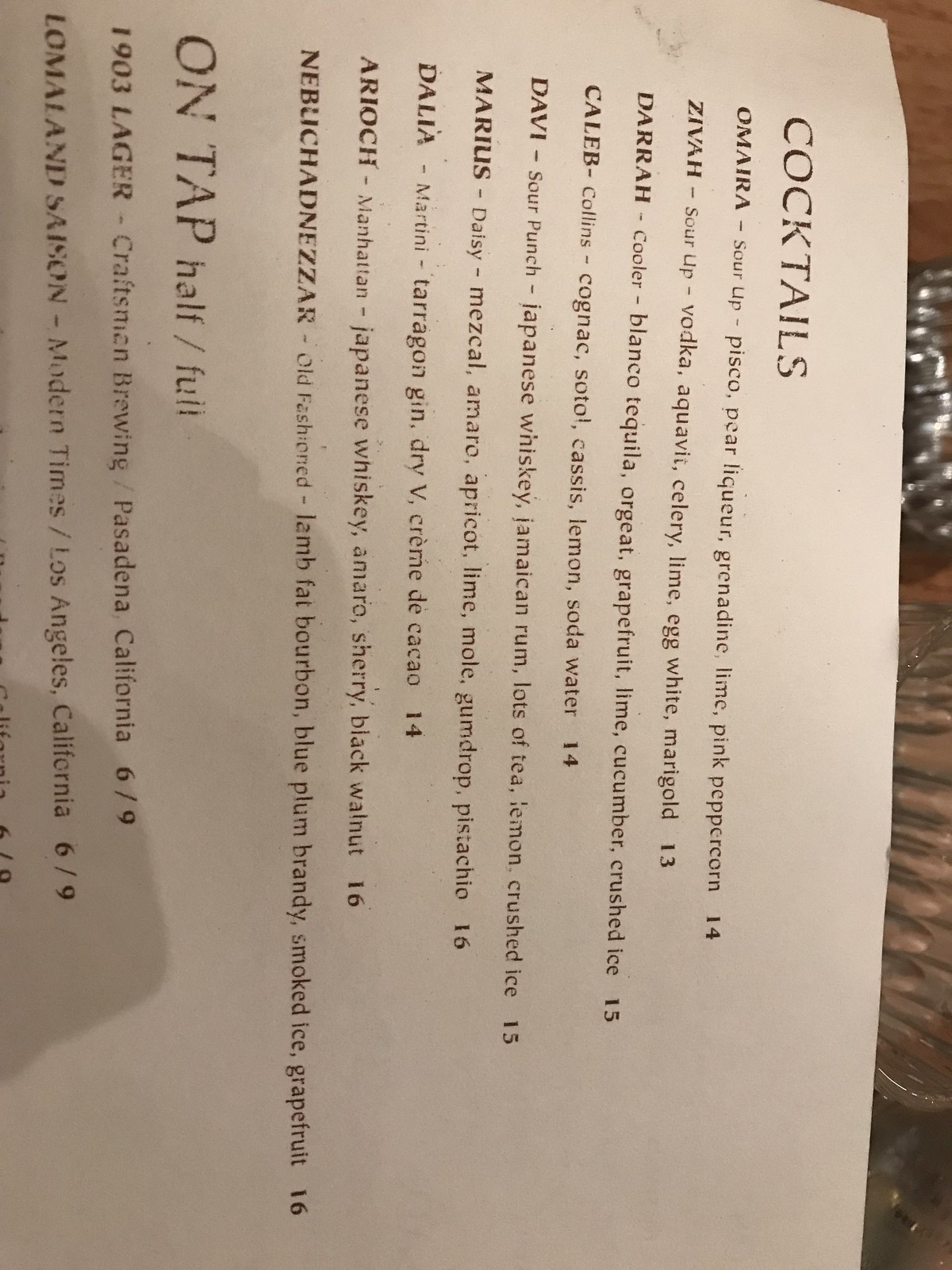This photograph, currently rotated requiring you to turn your head to the right to view it correctly, captures a white piece of printer paper with black text. The paper appears to be part of a menu, as indicated by the structure and content. The portion of the menu that is visible primarily lists cocktails, each name printed in bold with their ingredients and prices, avoiding specific details but including items named Omara, Ziva, Dara, Caleb, Davi, Marius, Dahlia, Ariok, and Nebuchadnezzar, with prices ranging from $13 to $16.

In addition to the cocktail list, the bottom portion of the visible section mentions an "on tap" section, referring to beverages on draft. However, the complete details of this section are obscured as the photograph only shows the top half of the paper.

Behind the paper, a shadow—likely that of the phone used to take the photograph—can be seen, adding depth to the image. The background of the photograph, seen in a narrow strip above the printer paper, appears to be a mix of brown wood and some unidentified silver objects, enhancing the casual, possibly rustic, ambiance suggested by the menu.